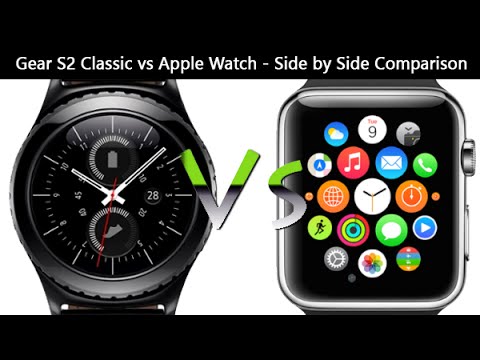This image presents a detailed side-by-side comparison of the Gear S2 Classic and the Apple Watch, depicted within a screenshot of a video thumbnail. At the top, written in white text against a wide black bar, it reads "Gear S2 Classic vs. Apple Watch Side-by-Side Comparison." A thinner black bar runs along the bottom of the image. The central white background features near its top the letters "VS" in a striking green and silver gradient.

On the left, the Gear S2 Classic is showcased. The watch has a black casing and an analog face displaying the time as approximately 10:08, with white hands and numerals, and distinctive white dash marks. A slim red second hand adds a touch of color.

On the right, the Apple Watch is displayed with its iconic rectangular face dominated by various colorful circular app icons, such as messaging, calendar, and photos. The watch includes a small, silver round dial positioned on the right side.  

The overall layout against a clean white background highlights the contrasting designs and functionalities of these two sophisticated smartwatches.